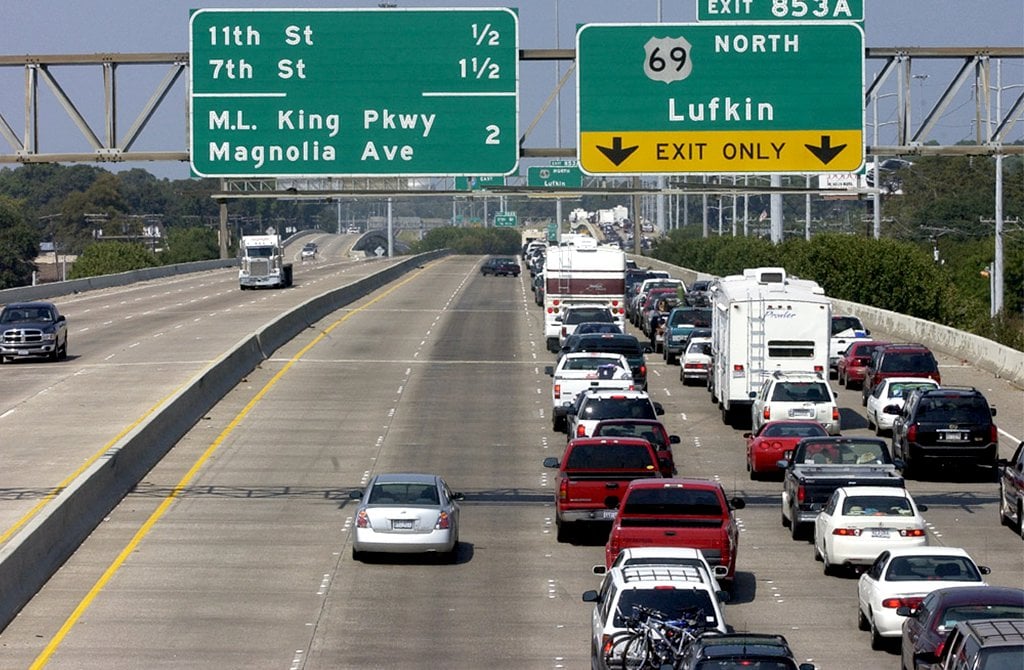The image depicts a bustling highway scene with dense traffic. On the left-hand side, two lanes are conspicuously clear except for two cars, while the three right-hand lanes are jam-packed with vehicles in bumper-to-bumper traffic. This congestion is likely due to the nearby signage indicating that these lanes are directed towards Exit 853A for Highway 69 North to Lufkin, marked with "Exit Only." A large green sign above the crowded lanes reads details of the exits, specifying 11th Street in half a mile, 7th Street in one and a half miles, and ML King Parkway and Magnolia Avenue in two miles. The opposite lanes, divided by a median, appear sparsely populated, with a few vehicles traveling freely amidst the backdrop of dense green trees. The photograph seems to be taken from an elevated vantage point, possibly from atop a tall truck, offering a comprehensive view of the highway and the detailed dynamics of the traffic below, which includes multiple RVs, trucks, and cars of various colors.